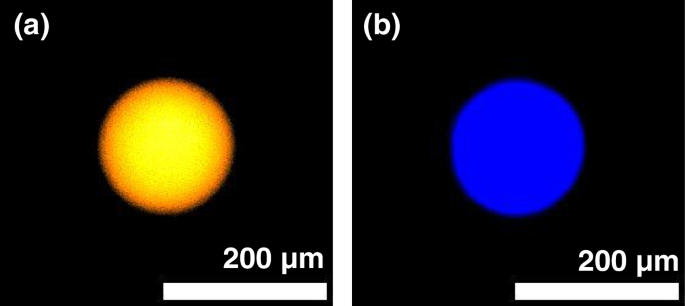The image is divided into two black-backgrounded squares, each depicting a circular object. The left square, labeled "(a)" in white text in the top left corner, features a centrally located yellow circle with an orange edge, resembling the sun. The right square, labeled "(b)" in white text in the same position, displays a central blue circle. In both images, the bottom right corner indicates a scale of "200 nm" (nanometers), and directly beneath this scale, there is a long white rectangular bar, representing the 200 nm length. The overall appearance suggests microscopic photographs displaying objects smaller than 200 nanometers in diameter.